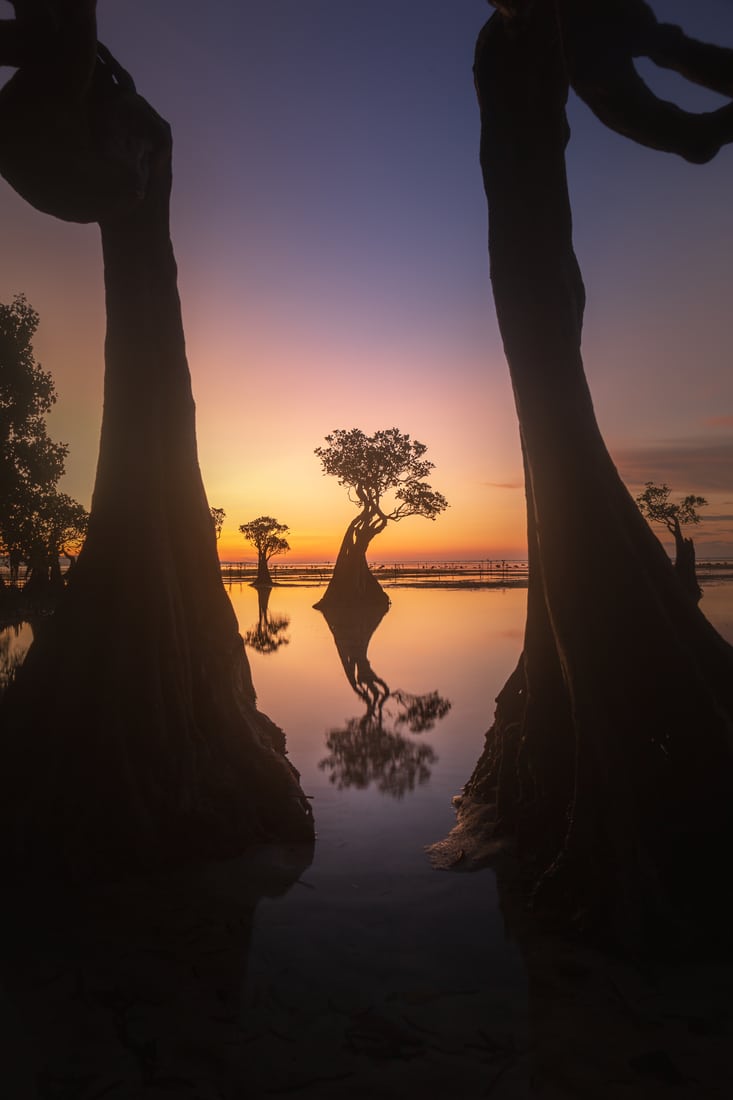This vertically aligned rectangular image captures an enchanting evening scene in a tranquil wetland. The sun has just set, casting a serene glow across the landscape. The sky exhibits a beautiful gradient, with a dark bluish-gray hue at the very top that transitions smoothly into dark purple and eventually into a vivid orange near the horizon, enhanced with layers of wispy pink and orange clouds. 

Dominating the foreground are two prominent tree trunks emerging from the still, dark charcoal-gray waters, their bases wide and sturdy, tapering as they rise and then curving gracefully at the top, almost giving the impression of hands reaching out. These curious trees create a natural frame through which the viewer is drawn deeper into the scene. 

In the background, other similar trees with large bases and thin, curvy trunks extend upwards, crowned with leaves. These trees reflect perfectly on the mirror-like surface of the water, further enhancing the calmness and surreal quality of the setting. The entire composition captures a timeless moment, rich with the reflection of the glowing sunset and the delicate interplay of light and shadow upon the water and in the sky.